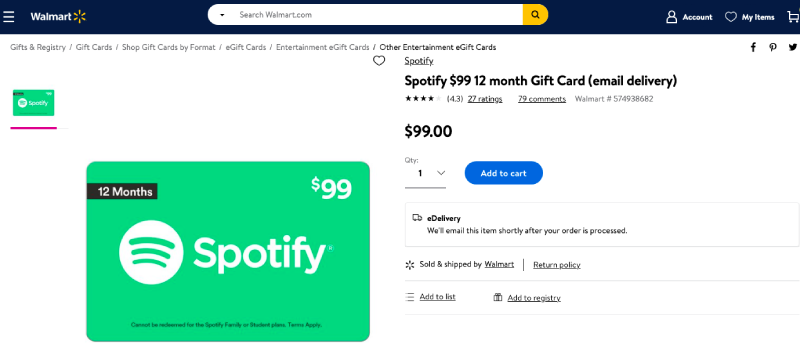The image displays a webpage from Walmart's website, featuring various elements of the online shopping interface. At the top, the Walmart logo is prominently shown alongside the website's navigation bar where one can search "walmart.com". The options for "Account," "My Items," and the shopping cart are also visible. Below these, there are links for "Gifts & Registry", "Gift Cards", "Shop Gift Cards by Format", "E-Gift Cards", "Entertainment E-Gift Cards", and "Other Entertainment E-Gift Cards".

Further down, the page showcases a specific product: a "Spotify $99 12-Month Gift Card" with email delivery. The product has received a 4-star rating based on 22 reviews and has garnered 79 comments. The price of the gift card is $99, and the customer has already added one to their shopping cart. 

To the right of the product, there is an image of a truck with the information "E-delivery: We will email this item shortly after your order is processed." It also mentions that the item is sold and shipped by Walmart and includes details on their return policy. Additional options to "Add to List" and "Add to Registry" are also provided.